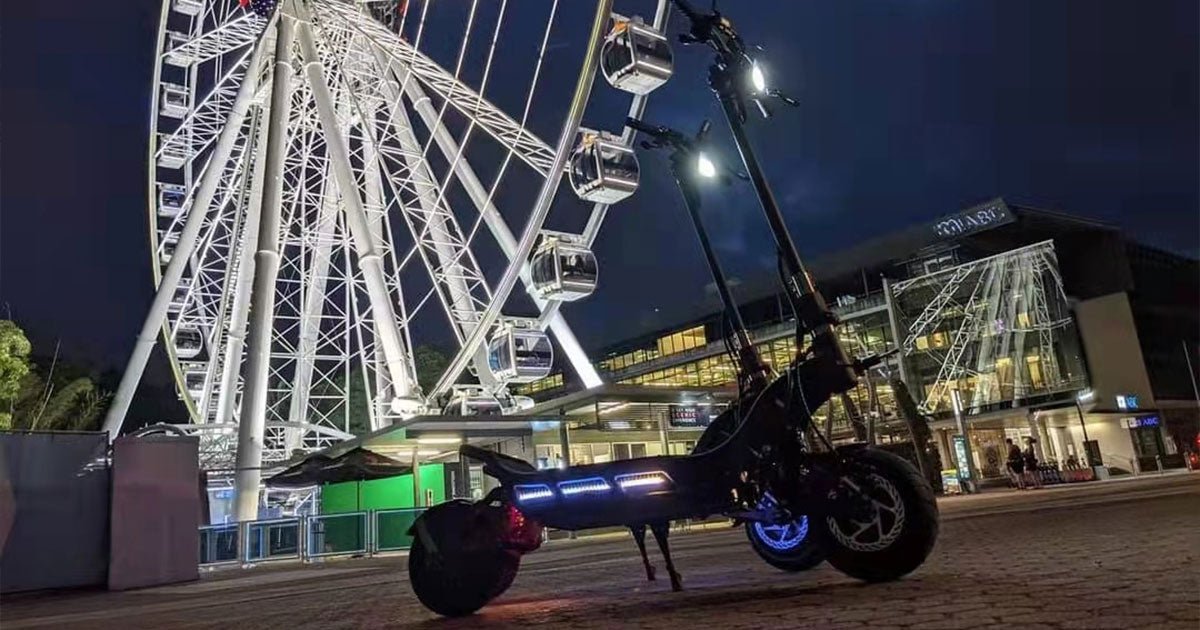The image captures a nighttime scene prominently featuring a towering white Ferris wheel photographed from a low angle, giving a sense of looking up from the ground. This Ferris wheel, set against a dark, evening sky, glows with lights that accentuate its structure. In the foreground, two black electric scooters with illuminated wheels are parked next to each other on a walkway with a honeycomb pattern. The scooters are positioned upright on their kickstands, ready for use. Off to the right side of the image is a large, well-lit building with multiple floors, providing a contrast to the otherwise darker surroundings. Additionally, a vividly lit green wall beside the Ferris wheel stands out prominently. The overall scene combines elements of modern urban transportation and entertainment amidst an established architectural setting.